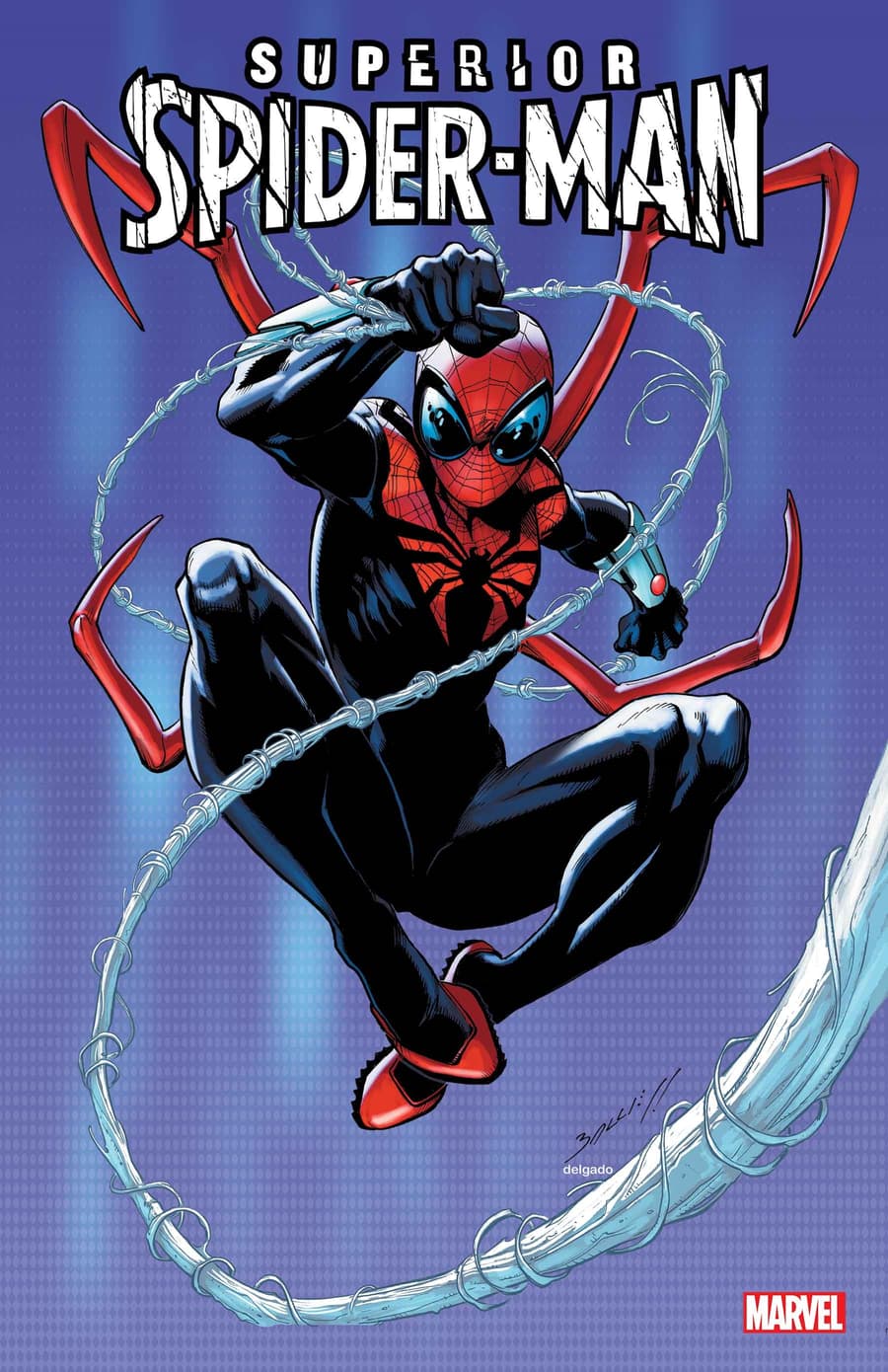The image is a detailed illustration of the front cover of a "Superior Spider-Man" comic book. Dominating the center, Spider-Man is depicted in a dynamic pose with his iconic suit, which features a darker blue and red color scheme than usual. His suit has large, reflective black eyes that suggest he's intensely focused on something, and a prominent spider logo on his chest. Spider-Man's legs are notably muscular and well-defined, with kneecaps and calves clearly visible, and he wears distinctive red shoes.

Intricately intertwined webbing is seen looping from his right hand, wrapping around his body, and extending across the cover, adding a sense of motion and energy to the scene. Notably, Spider-Man has four spider-like mechanical appendages protruding from his back, curving around him as if in a protective manner. His surroundings feature a gradient background that transitions from a deep blue at the top to a lighter blue at the bottom, with a subtle pattern of small squares and white accents throughout.

The top of the cover prominently displays the title "Superior Spider-Man" in bold white letters, and a red box in the bottom right-hand corner contains the Marvel logo. The overall composition is energetic and striking, with a purple hue subtly enhancing the background, making Spider-Man the unmistakable focal point.